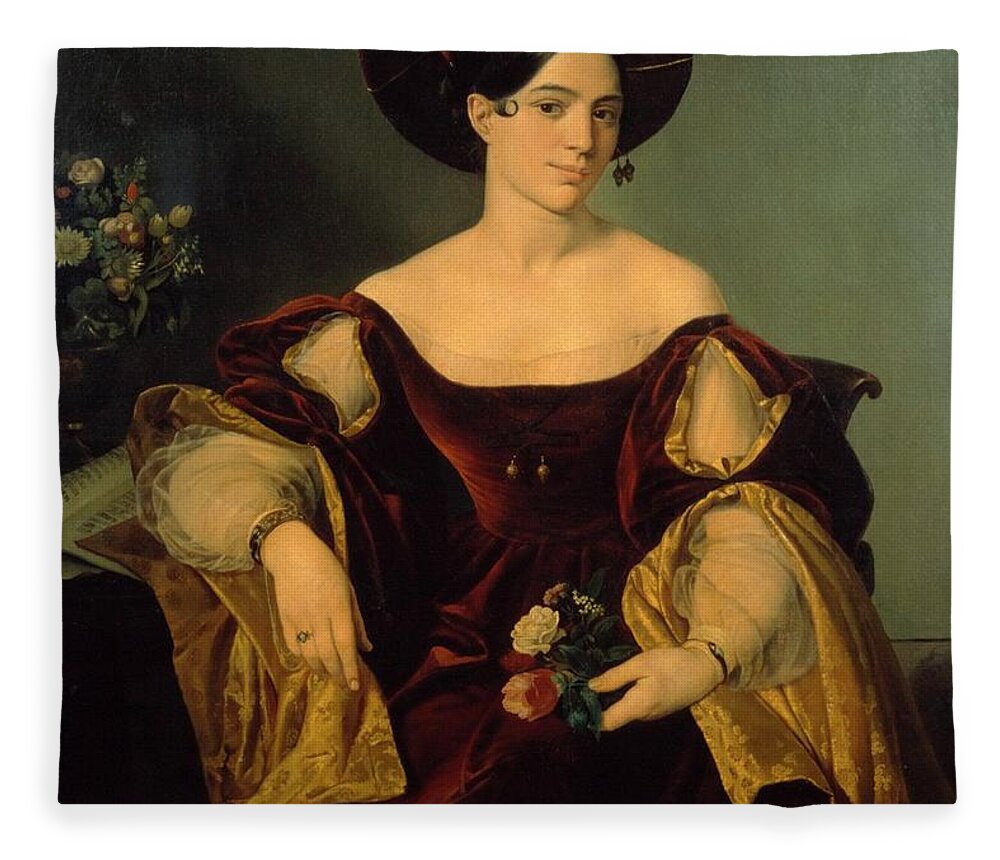This detailed Renaissance-style oil painting portrays a noblewoman seated in an opulent indoor setting. She dons an elaborate dark crimson velvet dress with white lace trim and sheer, transparent sleeves. Gold accents embellish her attire, including a blanket-like drape with a gold pattern. Her dark hair is partly obscured by a large, brimmed maroon hat adorned with dangling ornaments, possibly feathers or jewelry. She gazes coyly towards the viewer and holds a small bouquet of pink and white roses in her left hand, while her right hand, adorned with a ring, rests on a dark wooden chair. A table on her right supports a white book and more vibrant flowers in shades of red, yellow, and green. The background is a light gray, contrasting the dark blue and black hues that frame her chair, and suggesting an air of elegance and serenity. The painting’s textured details evoke the rich tapestry style of the 1600s, typical of Renaissance portraiture.